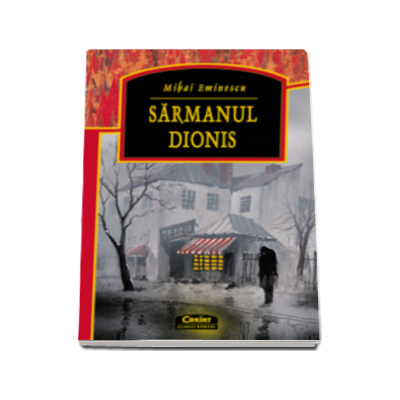The image depicts a photograph of a book standing upright against a stark white background. The book, titled "Sarmanul Dionis," features the author's name, Mikai Eminesu, in yellow text at the top, although it's somewhat blurry. The main visual on the cover is a grayscale illustration of a person standing outside near buildings with dimly lit interiors, suggesting a nighttime or winter setting. These buildings include homes and businesses, one of which has a white and red striped awning. The book also has a prominent red and orange border, adding a burst of color to the mostly muted grayscale cover. The text on the book is horizontal, with "Sarmanul Dionis" displayed prominently in the upper half around a black box. Despite some blurriness in the text details, the book's cover is well-defined and detailed, implying it could be part of a book website's catalog.